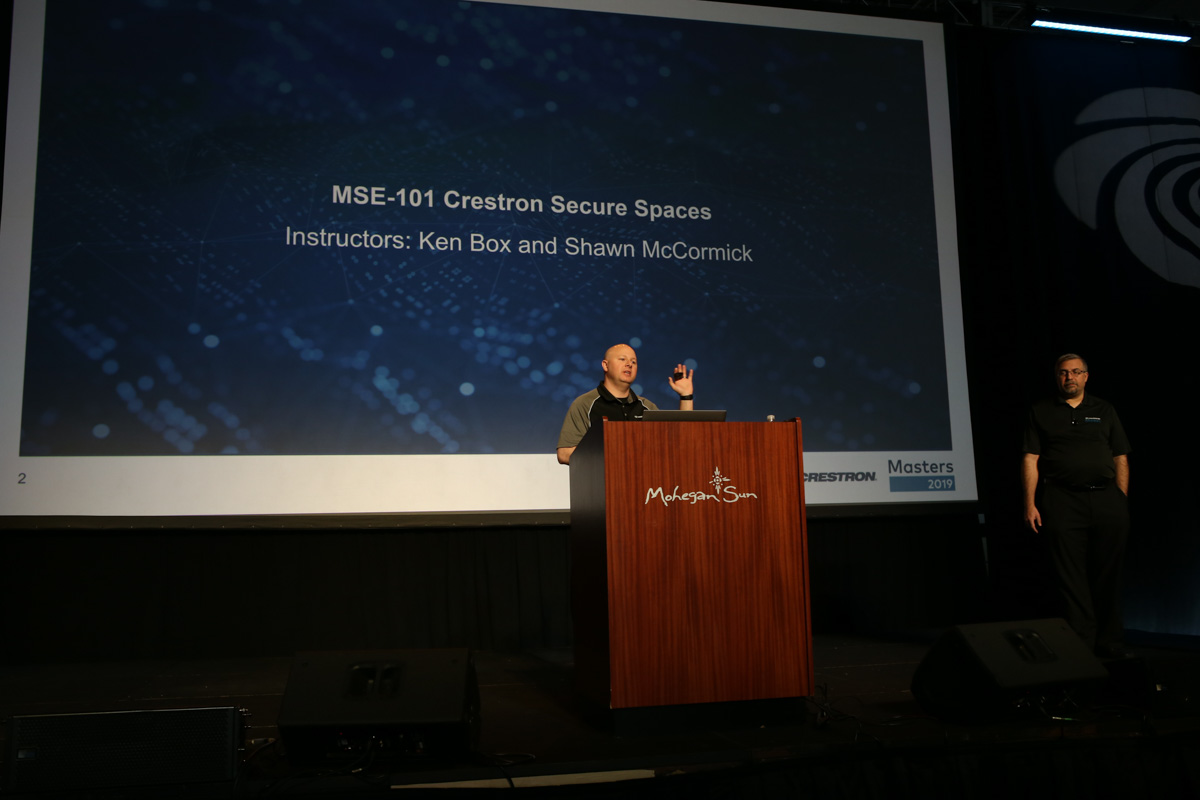The photograph depicts a man, centrally positioned, standing at a podium in a dimly lit conference room. He is white and bald, wearing a black and gray shirt, and has a wristwatch on his left hand, which holds a small black box aloft. The podium he stands behind features the logo "Mohegan Sun," suggesting the setting is within this casino's conference or hotel facilities. 

To the right of the man, another individual is visible, sporting a short-sleeved shirt with a logo and glasses. Behind the main speaker, a large screen displays the text "MSE-101 Creston Secure Spaces," identifying the instructors as Ken Box and Sean McCormick. In the bottom right corner of the screen, the words "Masters 2019" are clearly visible. The background of the screen consists of a blue abstract image. The room's darkness is alleviated by a band of light in the top right-hand corner, possibly from a tube light. The atmosphere and arrangement of elements hint at an educational or professional presentation.